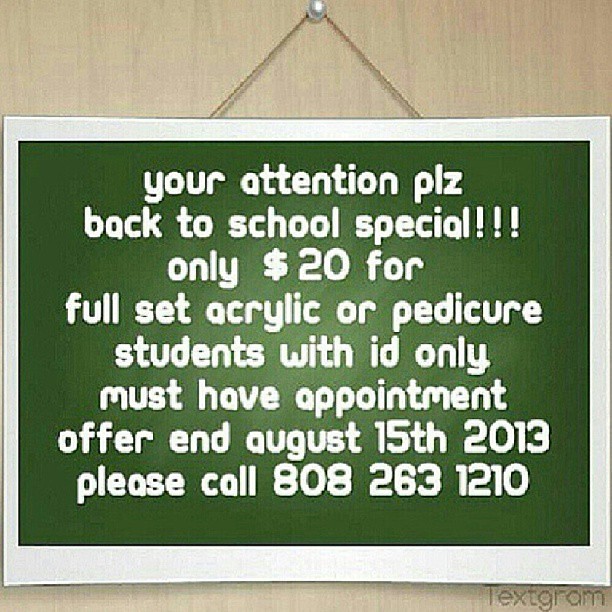The image depicts a clipart-style sign hanging on a wooden wall or door, secured by a string connected to a pearl push pin or nail. The sign features a white border with a green background and white text. The text, slightly pixelated, reads: "Your attention please" (spelled "PLZ"), followed by "Back to school special!!! Only $20 for a full set of acrylic or pedicure. Students with ID only. Must have appointment. Offer ends August 15, 2013. Please call 808-263-1210." At the bottom right corner, there's a faint black text that says "textgram."